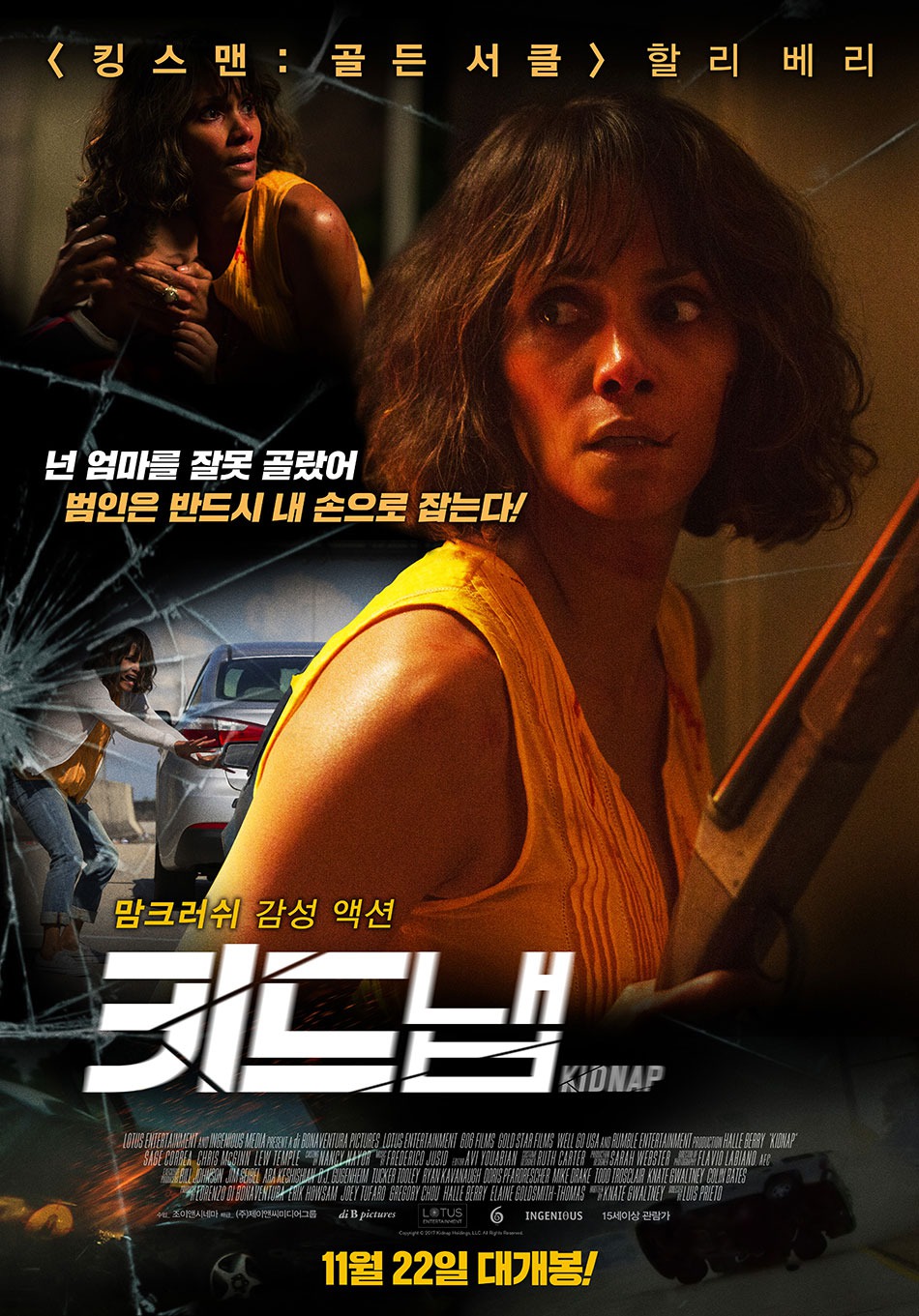This is a detailed movie poster primarily featuring an African-American woman who appears distressed and frightened. Most of the text on the poster is written in Korean, with the only discernible English word being "kidnap." The main image showcases the woman in an orange sleeveless top, which has some blood on the collar, holding what seems to be a brown shotgun. She has a cut on her upper lip and is looking off to the side. In one corner, there is a smaller inset of the same woman, seen from behind a silver or gray sedan, looking panic-stricken and backing away as if she's trying to stop another vehicle. Another small image depicts the woman with her hand over a young girl's face, attempting to keep her quiet, indicating a tense situation. Additional scenes include a cracked windshield and a vehicle flipping, hinting at dramatic, action-filled sequences in the movie. The entire composition of the poster, with its montage of scenes and vivid character portrayal, strongly suggests a thriller centered around a kidnapping.